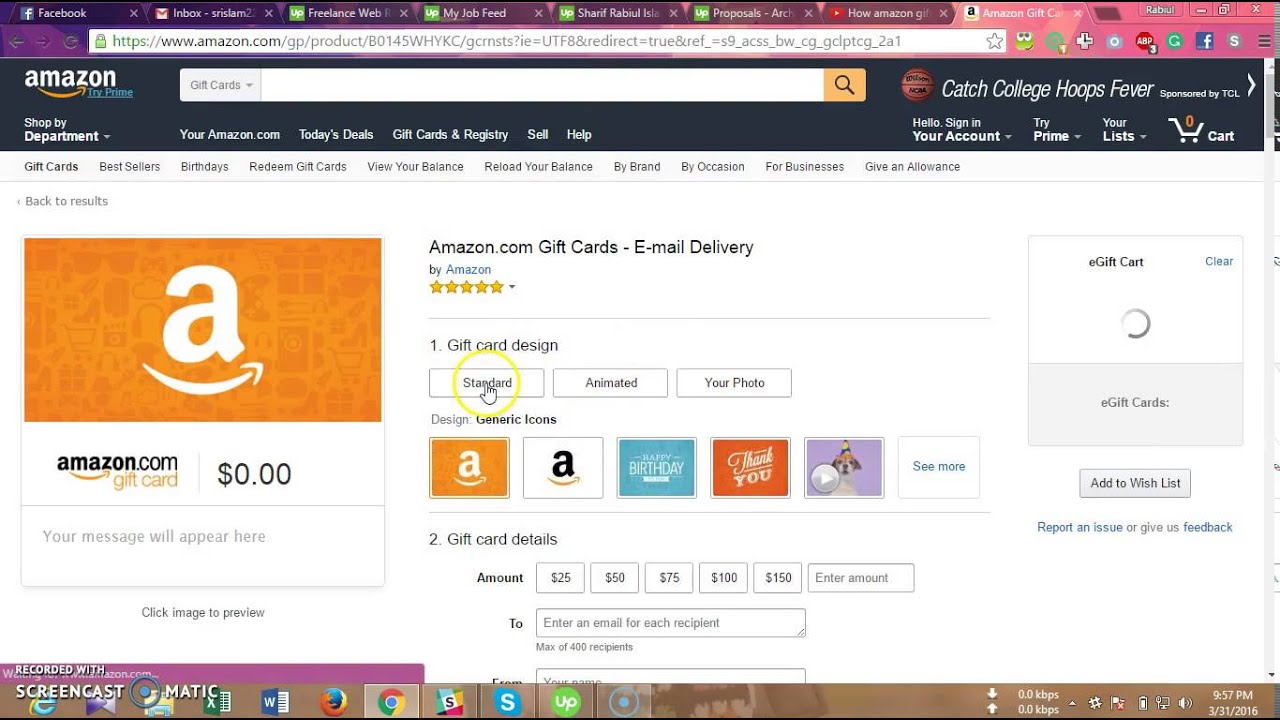Captured on an Amazon page, the browser displays several open tabs in the order: Facebook, Inbox, Freelance Web, My Job Feed, Sharif Rabiel, Proposals, and a YouTube video titled "How Amazon Something". The Amazon page features an advertisement adjacent to the search bar reading, "Catch College Hoops Fever," accompanied by a basketball graphic on its left.

Displayed prominently, the page is set on the gift card section, marked by categories such as Best Seller, Birthdays, Redeem Gift Card, View Your Balance, Reload Your Balance, By Brand, By Occasion, For Businesses, and Given Allowance. Below these categories, the heading states "Amazon.com Gift Card - Email Delivery by Amazon," highlighting it as the number one gift card design.

Three gift card design options are presented: Standard, Animated, and Your Photo. The Standard option is highlighted with a yellow circle around it. Beneath this, a description indicates the design style as "Generic Icons."